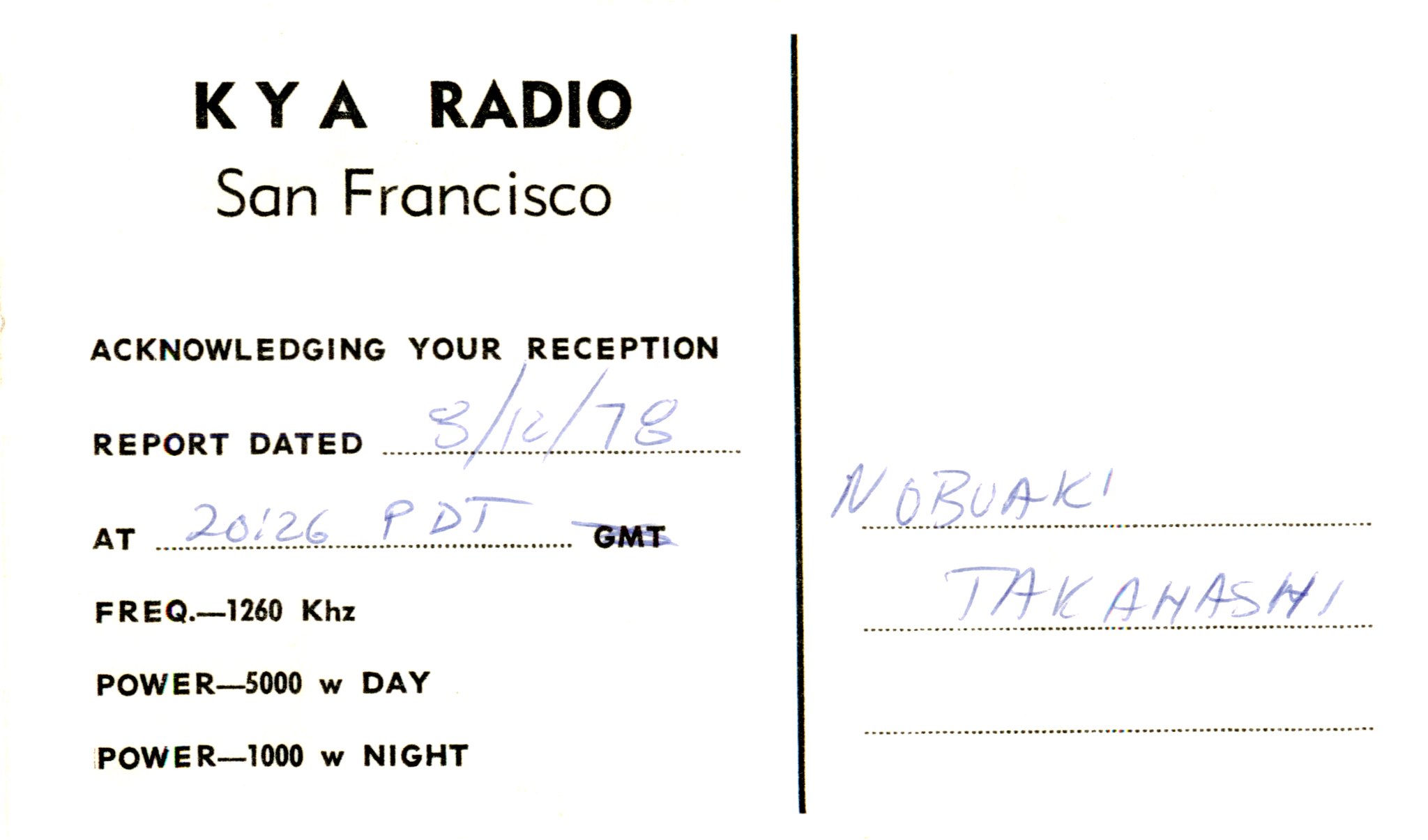The image depicts the back of a white postcard featuring printed and handwritten text in black and blue ink respectively. The postcard, which is white with black lettering, is divided into two sections by a vertical black line running centrally down the middle. The left section prominently displays "KYA Radio" in bold, centered text, followed by "San Francisco," which is not bolded but also centered. Below this, it states "Acknowledging Your Reception" and "Report Dated," with the latter accompanied by a handwritten date in blue ink, "8-10-78." Below the date, it reads "At," followed by "2026 PDT," written in the same blue ink. Additionally, there is text indicating the station's frequency as "1260 kHz" and power information as "5000 W day" and "1000 W night." On the right section of the postcard, which contains three lines of handwritten text in blue ink, the name "Nobuaki Takahashi" is written in print. The details emphasize the acknowledgement of a reception report by KYA Radio in San Francisco.